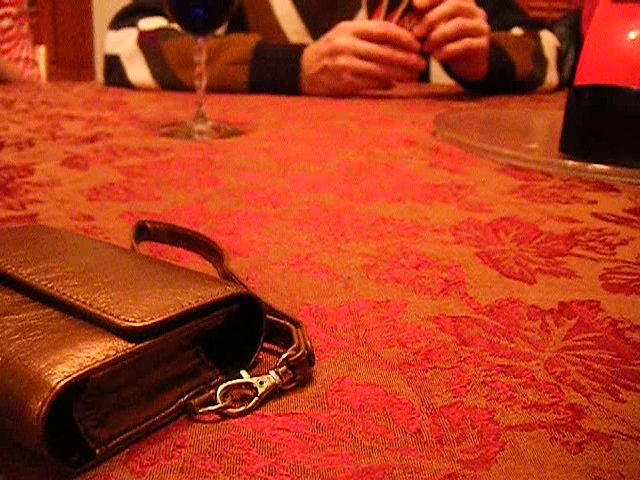In this indoor photograph taken at a shop, the focal point is a tabletop covered with a satiny, floral tablecloth featuring intricate, red and orange patterns of flowers and foliage. Resting on the table is a small, brown, fold-over, wallet-style clutch purse with a clip-on, skinny brown leather wristlet. Across the table, a person is partially visible with their forearms resting on the tablecloth. In front of them sits a glass of red wine, marked by a distinctively twisted stem. The individual is wearing a brown, black, and white striped sweater and appears to be holding playing cards. The combination of the tablecloth’s vivid texture, the elegant clutch, and the casual yet refined atmosphere conveyed by the wine and cards underscores a sense of cozy sophistication.